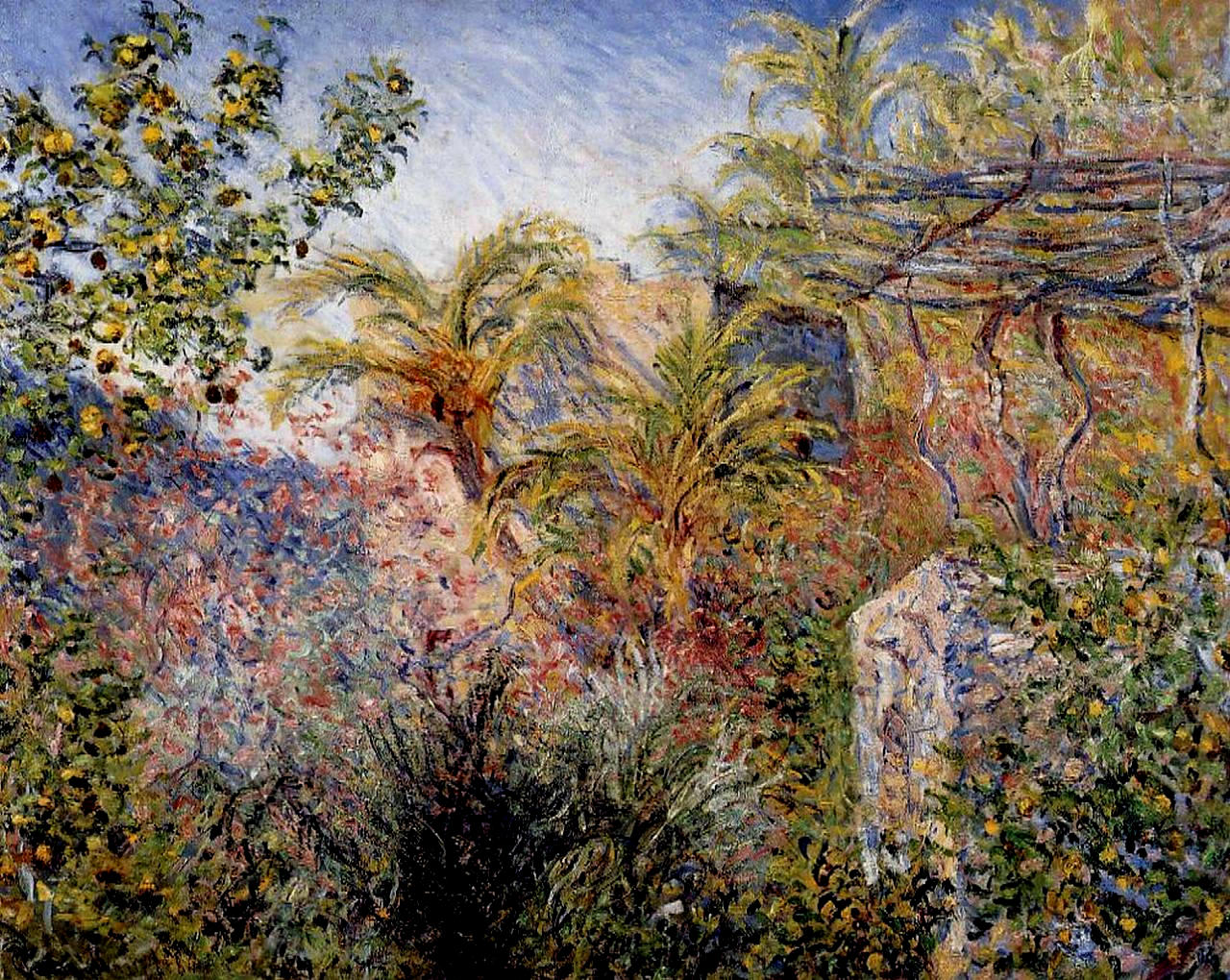In this vibrant painting of an outdoor garden during the daytime, a detailed scene unfolds, filled with varied flora and intricate elements. The foreground is dominated by a rectangular stone pillar surrounded by verdant plants adorned with bright orange flowers. To the lower center, a dark green bush adds depth to the lush garden setting. Left of the bush is a tree boasting yellow flowers, while the middle of the scene features a series of plants in shades of red and blue, further enhancing the garden's rich palette. Palm trees dot the midground, their distinctive leaves painted with sweeping brushstrokes. On the right, an intricate wooden structure, reminiscent of latticework or a grill, stands out, decorated with dainty flowers nestled among vines. The rock below this wooden structure is a mosaic of colors, clearly identifiable in its natural form. The top right corner reveals more palm trees, juxtaposed against a serene blue sky filled with soft, white clouds. The left side of the painting showcases additional foliage, interspersed with flowers depicted as delicate dots of color. Overall, the painting captures a colorful and serene garden scene, blending detailed botanical elements with artistic brushwork to evoke a sense of peaceful nature.